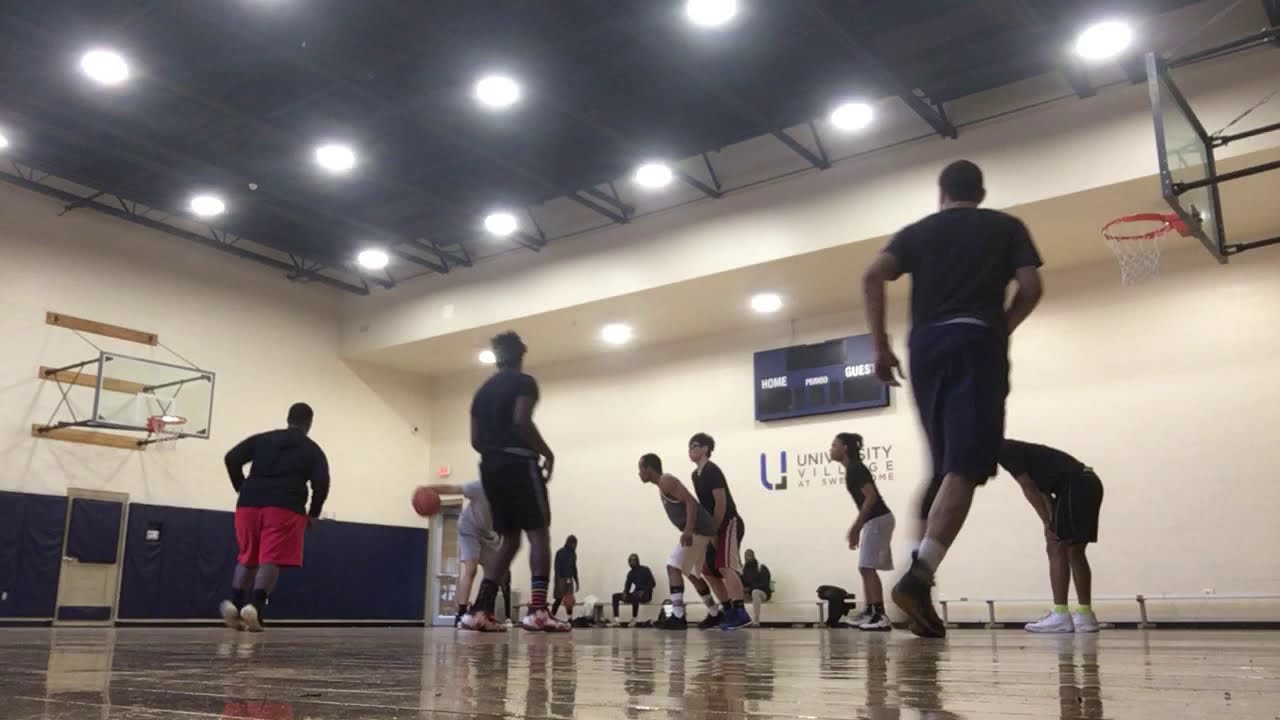The image captures an indoor basketball game at a gymnasium identified as University Village. The entire scene is dominated by a highly glossy wooden floor, so polished that it mirrors the players, making it appear as if they are walking on water. The composition is shot from a low, floor-level perspective, accentuating the lofty ceiling with its intricate steel girders and evenly spaced bright lights. The walls of the gym are mostly white, with sections of blue padding where the basketball hoops are mounted.

The gym is populated by eleven amateur players, distinguishable by their varied attire, which ranges from dark to brightly colored jerseys and shorts, and a mix of different colored sneakers. This lack of uniformity, along with the mixed ethnicity of the players, gives the impression of a casual pickup game rather than an organized team match. Near the center of the court, a man clad in dark clothing actively dribbles the basketball, drawing the attention of the others who seem ready to defend.

In the background, to the right, a scoreboard looms, displaying 'Home' and 'Guest' scores, and just beneath this, the words "University Village" are partially obscured by a standing player. Below the scoreboard is a bench where a couple of players are seated, and to the far left of the image is an exit door. The overall atmosphere is brightly lit, emphasizing the dynamic energy of the scene.